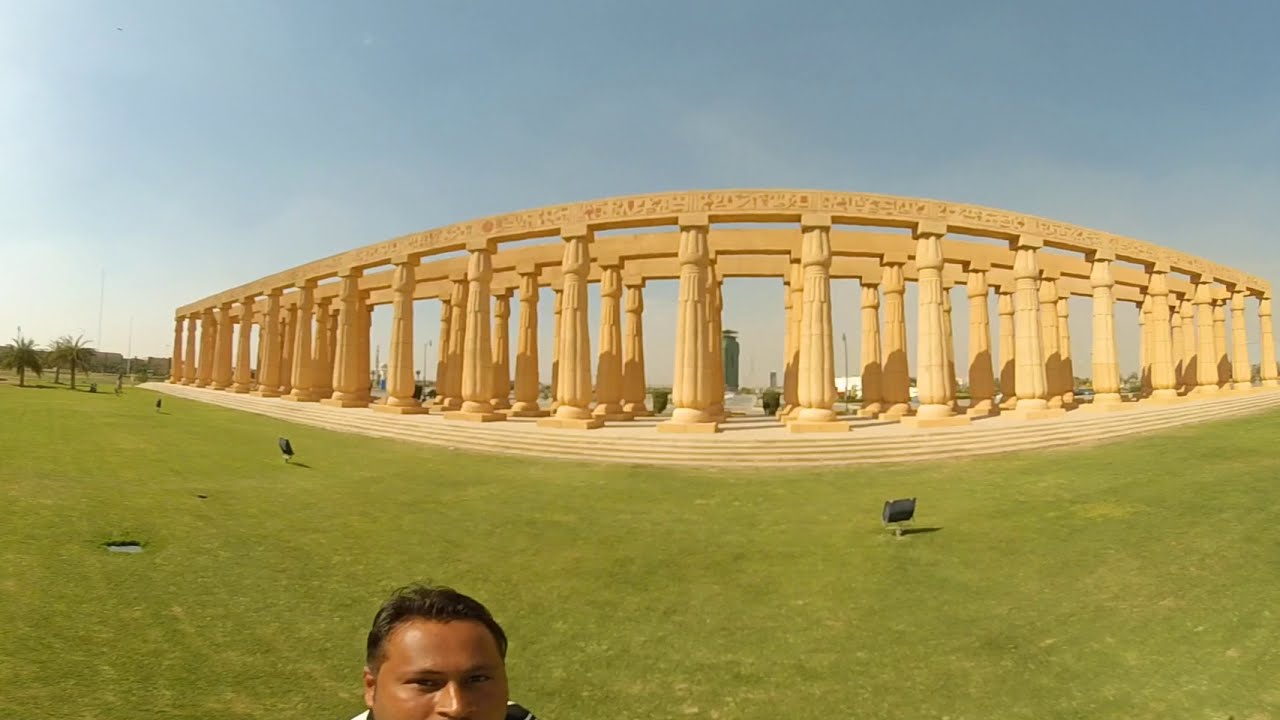In the foreground of the image, a man, likely of South Asian or Hispanic ethnicity with darker skin and short brown hair, is taking a selfie with a selfie stick. The photo captures him from the nose up. The background reveals a meticulously tended vibrant green lawn dotted with black spotlights, all pointing towards a grand structure. This historic monument features a series of six steps leading up to three rows of yellowish-cream, Greek-style decorative columns. The columns support an engraved beam at the top, though the details of the engravings are not clear. To the left edge of the image, several palm trees are visible against a light blue sky with scattered, muted clouds. The sun is illuminating the scene, enhancing the overall brightness and clarity without being directly visible in the photo.